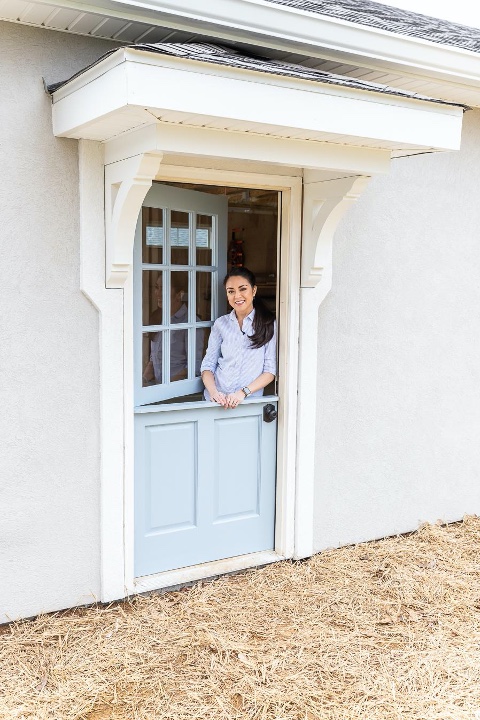In this image, a woman stands smiling in the center of a white building's doorway, exuding happiness. The building features a distinctive blue split door, with the top half open, and is framed by ornate, white-painted wooden decorations. Black asphalt shingles cover the visible part of the roof, seen in the upper right corner of the photograph. The ground outside is scattered with straw, reminiscent of a barn or equestrian facility setting. The woman, dressed in a light blue button-up shirt, has dark hair pulled back in a ponytail and places her hands on the closed bottom half of the split door, looking directly at the camera.